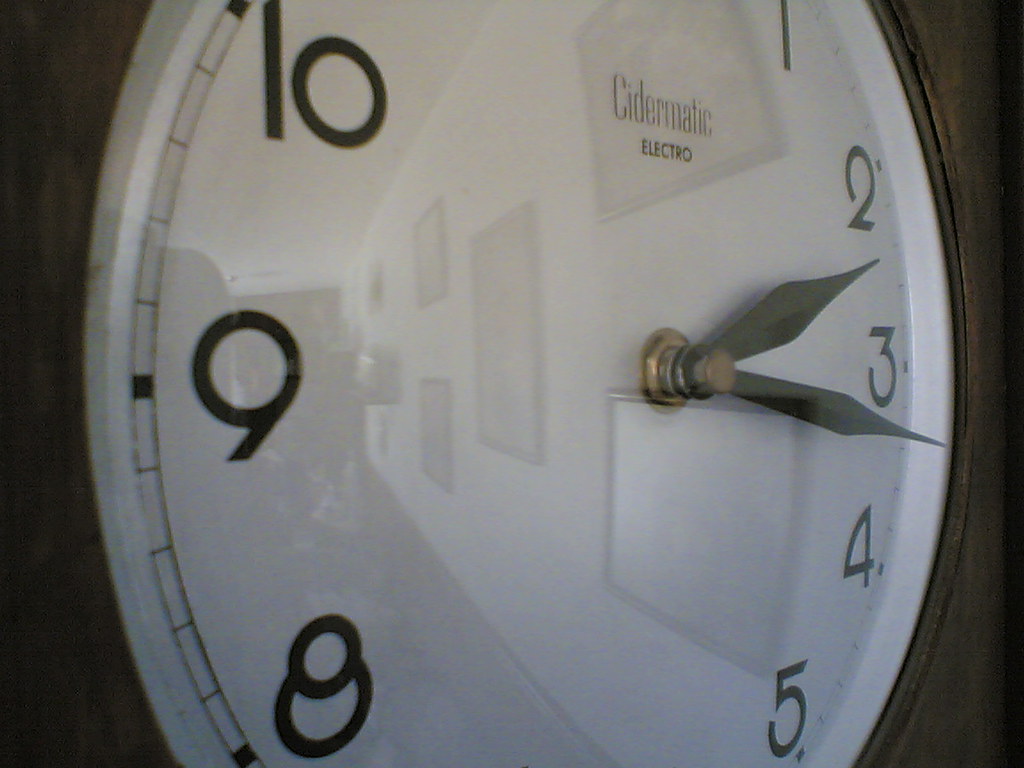The image shows an extremely close-up view of a circular clock captured in high detail, revealing much about its design and surroundings. The clock features a glass cover with a dark brown, almost wooden, circular frame. Its background is white, showcasing conventional black numbers from 1 to 12; however, due to the tight framing of the photo, only the digits 1, 2, 3, 4, 5, 8, 9, and 10 are visible, with other numbers such as 6, 7, 11, and 12 cut off. The black hands of the clock indicate a time of approximately 2:17. Above the hands in bold black lettering is the text "CIDERMATIC," and beneath that, in smaller black letters, it reads "ELECTRO." 

An interesting feature of the clock is the minute markers, represented by double lines around the outer edge, along with accompanying white squares. Due to the glass cover, a reflection of the room in front of the clock is visible. This reflection reveals a white wall adorned with at least six or seven framed pictures, as well as a table at the far end that holds many smaller pictures. Though the exact details in the frames are indistinct, the overall setting suggests a long room filled with decorative elements.